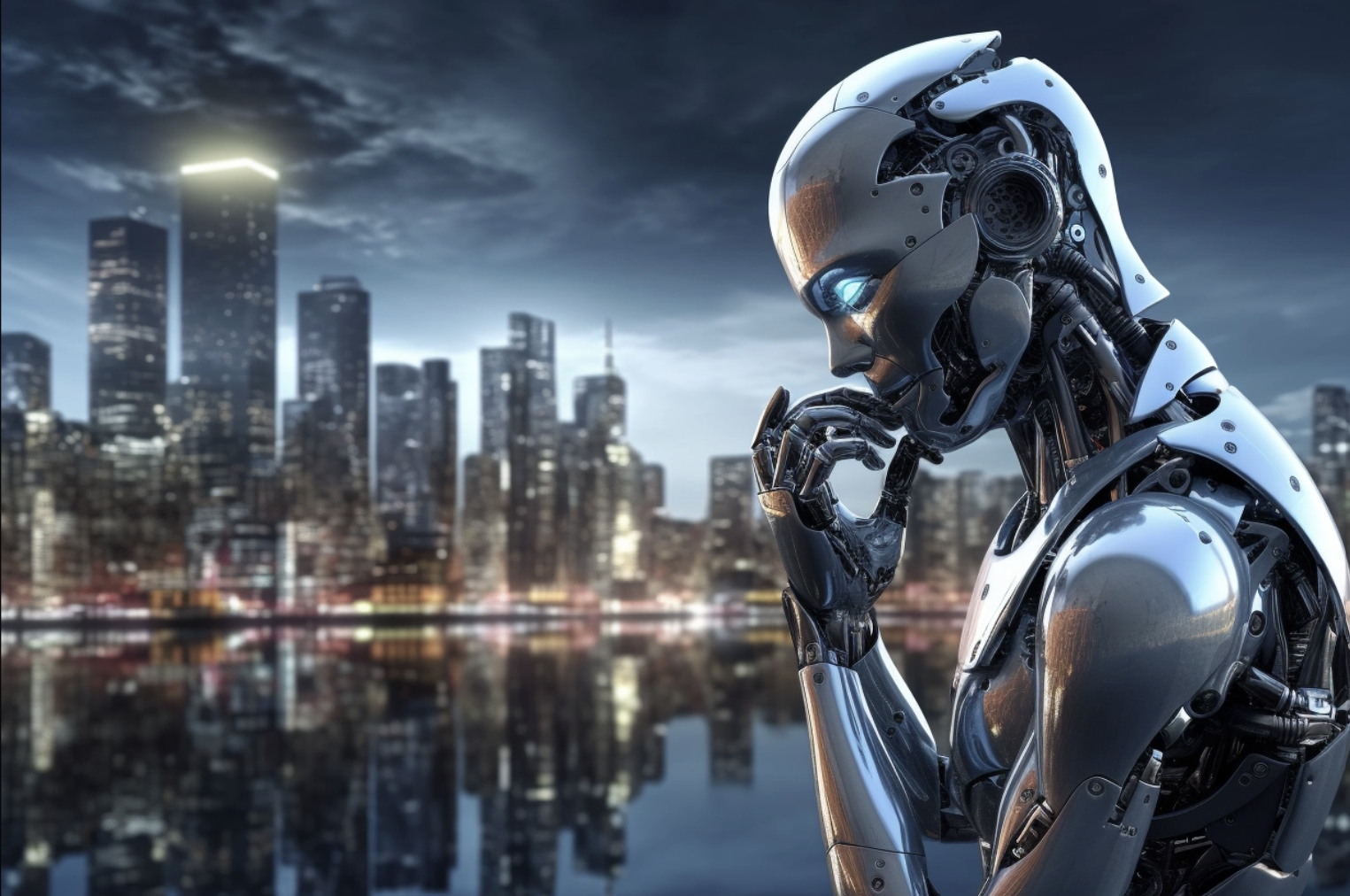A detailed 3D rendering depicts a futuristic scene featuring a human-like robot set against a backdrop of a modern city skyline. The rectangular image is twice as wide as it is tall. The robot, positioned prominently on the right side, is constructed from semi-glossy white panels that reveal intricate inner workings such as machinery, hydraulics, and cables. With humanoid facial features, including lips and a nose, its glowing light blue eyes stand out. In a contemplative pose, its head slightly tilted down, the robot's hand is raised to its chin, emphasizing a human-like gesture of thinking. The background showcases a serene large body of water, reflecting the cityscape, which is filled with towering skyscrapers adorned with yellow lights, under a dark blue, purple-tinged sky. The scene combines vivid technological details with an evocative atmosphere, blurring the lines between the mechanical and human realms.